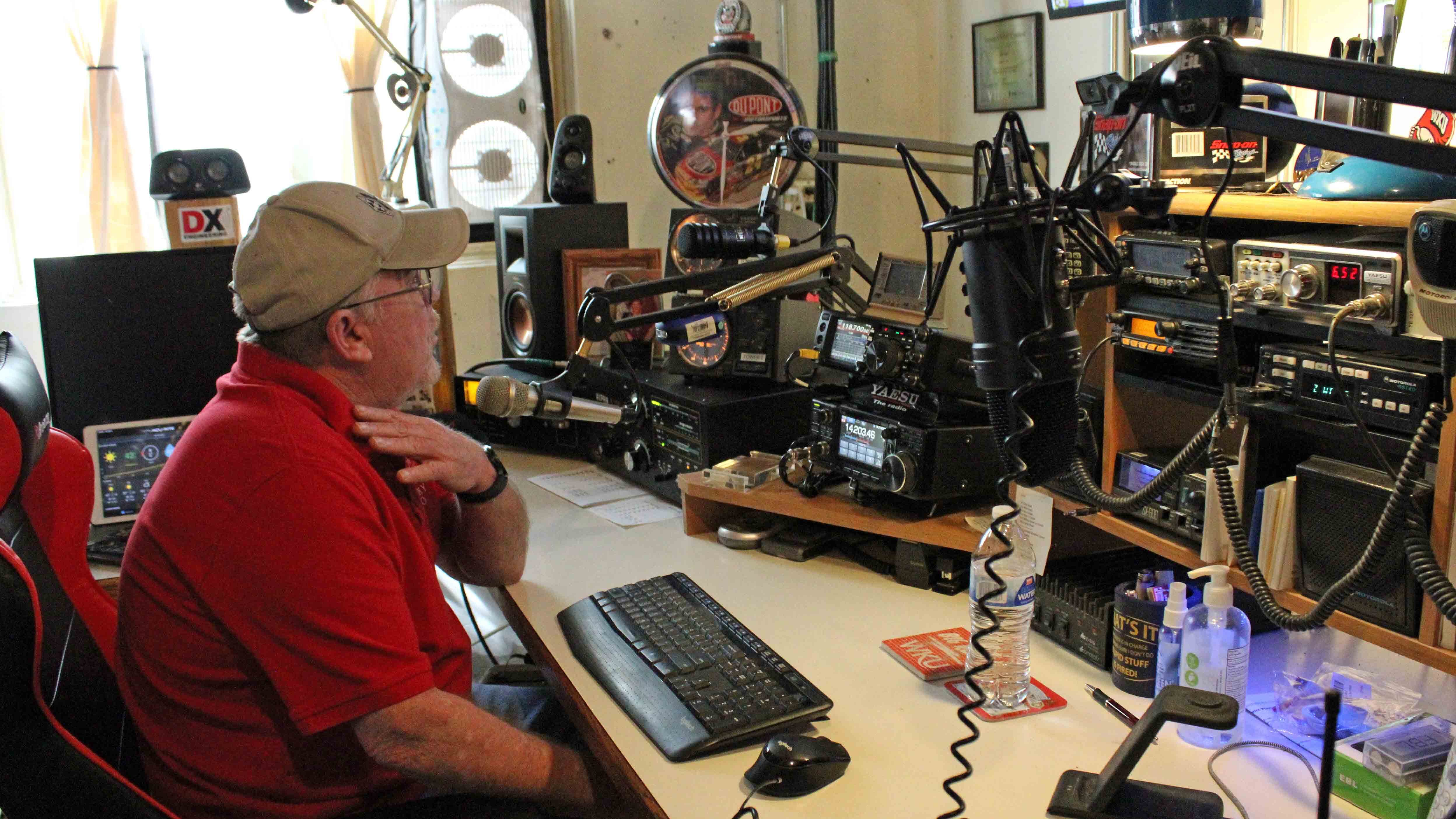In this image, we see an older man with glasses and gray hair, seated behind a long beige desk, facing slightly to the right. He is wearing a beige cap and a red short-sleeved polo shirt. He's sitting in a red and black gaming chair with his left hand on his neck and a black watch on his wrist. Directly in front of him on the desk are a black keyboard and mouse, and a silver microphone on an articulable arm positioned near his mouth. Numerous other pieces of communications equipment, including radios and sound machines, are cluttered across the desk and shelving on the right side. Black cables connect these devices, confirming his involvement in a sophisticated setup, potentially for radio broadcasting or similar activities. In addition, there are multiple stands with microphones on movable arms, and a distinctive DuPont NASCAR clock with a race car image is visible on the far wall. On the left side of the desk, there is a speaker and an iPad displaying weather information. Other items on the desk include a bottle of water, hand sanitizer, and what appears to be screen spray.